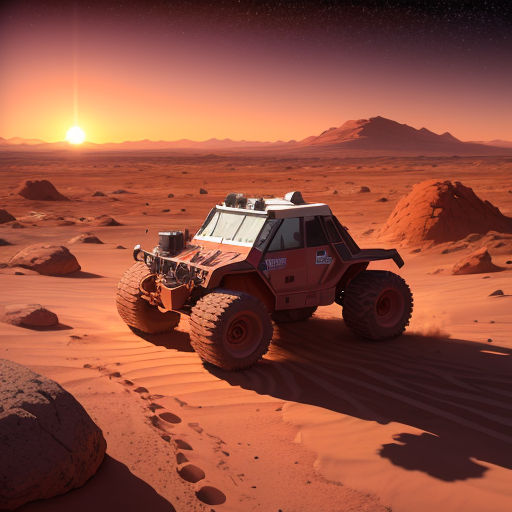The image portrays a detailed 3D scene that could either be a desolate desert on Earth or the surface of Mars, characterized by its reddish-orange sandy terrain. Prominently featured in the foreground is a rugged, dune buggy-like rover facing slightly to the left. The vehicle has large, all-terrain tires caked with orange dust, and its body is mostly brown with a white top. Distinctive markings, white writing, and logos can be seen on the sides. The rover is equipped with a three-piece windshield and side windows, and a black cylindrical object is located on the left side of the hood.

In the bottom left-hand corner of the image, a conspicuous large rock can be seen, with additional rocks scattered throughout the mid-ground. Notably, the sandy surface shows a trail of footprints leading from the front of the vehicle and veering slightly to the right out of the frame. The background is mostly flat with sporadic mounds and rocks.

Further in the distance, to the right, a large hill rises, while to the left, the horizon is marked by the Sun either rising or setting, casting a yellow, orange, and light purple hue across the sky, which darkens towards the upper right-hand corner. The overall scene is bathed in a soft, diffused light, adding to the eerie and desolate atmosphere of the landscape.